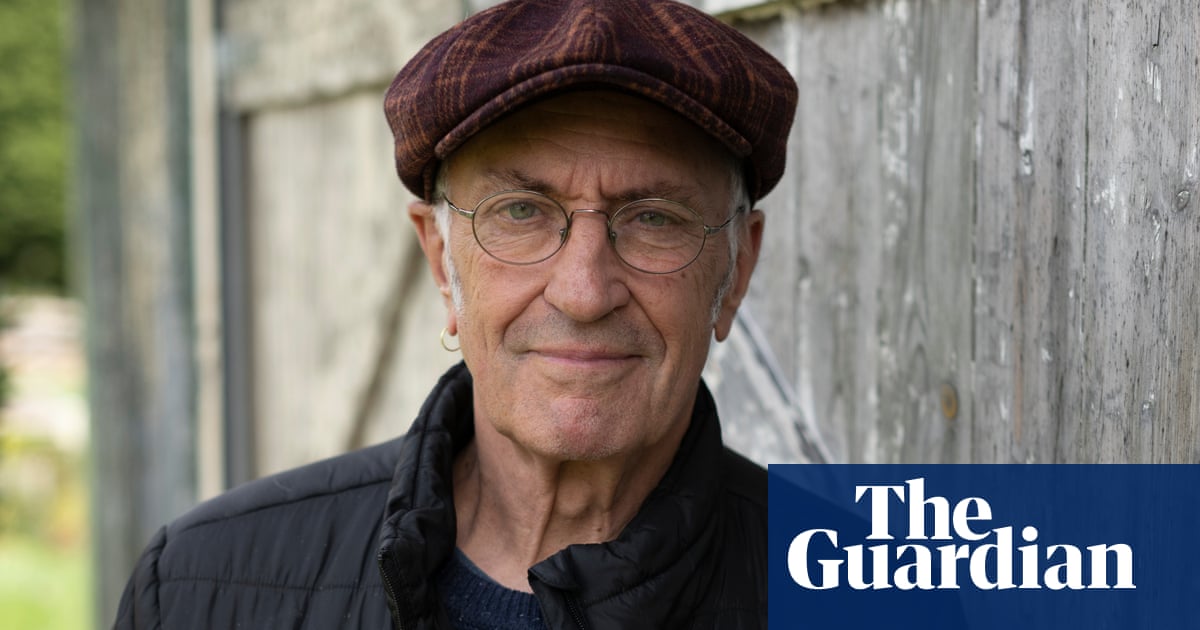The photograph, taken outdoors during the daytime, showcases a close-up of an older Caucasian man in front of a faded gray wooden barn with hints of green trees in the background. The man is central to the image, depicted from the shoulders up. He wears thin, circular gold-toned wire-framed glasses and a distinctive red and brown striped flat cap, reminiscent of a Gatsby hat. His short white hair peeks out in front of his ears, and he sports a gold hoop earring in his right ear. The man's grayish-green eyes are direct and intense, gazing straight into the camera with a subtle smile on his closed lips. He is dressed in a black jacket, layered over a black shirt. 

In the lower right-hand corner of the rectangular image, a transparent blue rectangle extends across an inch and a half to the left and half an inch upward before returning to the right. Within this blue rectangle, bold white text reads "The Guardian," indicating the image is an advertisement for the UK-based newspaper or magazine, The Guardian. The overall photo is clear and bright, with natural lighting enhancing the details.